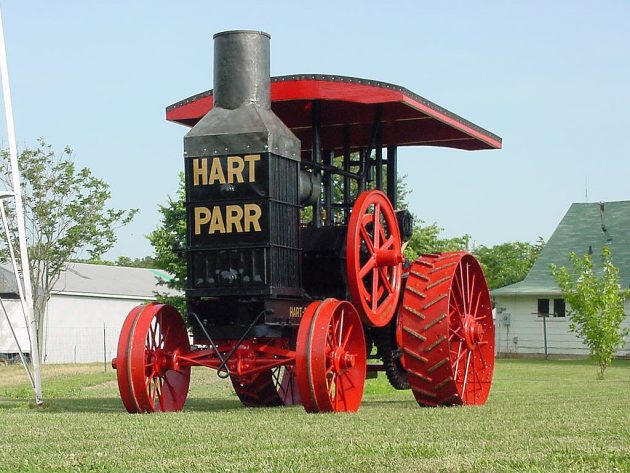Here is a refined and detailed descriptive caption for the image:

"This vintage coal-fired tractor stands as a testament to industrial ingenuity. Dominated by its mostly black coal burner and towering smokestack, it exudes a rugged charm. The operator's area is painted black, framed with iron squares reminiscent of windows. The roof, also black, reveals a striking red underbelly. A massive red wheel, likely forged from cast iron or steel, commands attention on the side, complemented by imposing red-painted rear tractor wheels. The front wheels, smaller yet similarly painted red, add to its robust appearance. The name 'HARTPARR' is emblazoned in gold on the front, adding a touch of elegance. This impressive machine is set against a backdrop of a neatly manicured yard with newly planted trees. A picturesque white house, featuring a Cape Cod roof, and a white warehouse or shop can be seen in the distance. The clear blue sky and bright sunshine enhance the scene, bringing every detail of the red and black tractor into sharp focus. This historical tractor, likely a centerpiece at a political event, symbolizes the hopes of the candidates standing beside it."